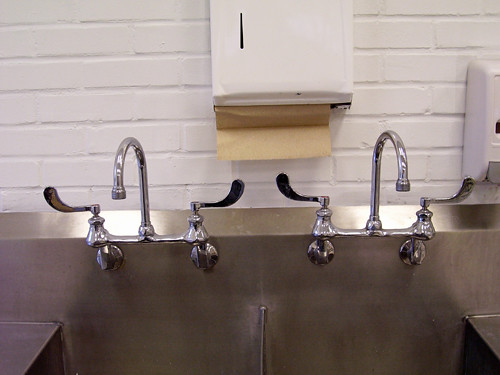The image shows a close-up view of a large, stainless steel sink situated in what appears to be a commercial or industrial kitchen. The sink, made entirely of stainless steel, is divided into two deep wells, each equipped with a separate set of hot and cold water faucets featuring large black handles. The sink's surface extends horizontally on both sides, forming sloped, flat pieces designed to drain water back into the basin. 

Mounted on the white brick wall behind the sink, there is a white metal paper towel dispenser in the center, dispensing brown industrial-style paper towels. Just visible on the right edge of the image is a white soap dispenser with a grey push lever. The setup suggests a highly functional, utilitarian space designed for heavy-duty cleaning and sanitation tasks.